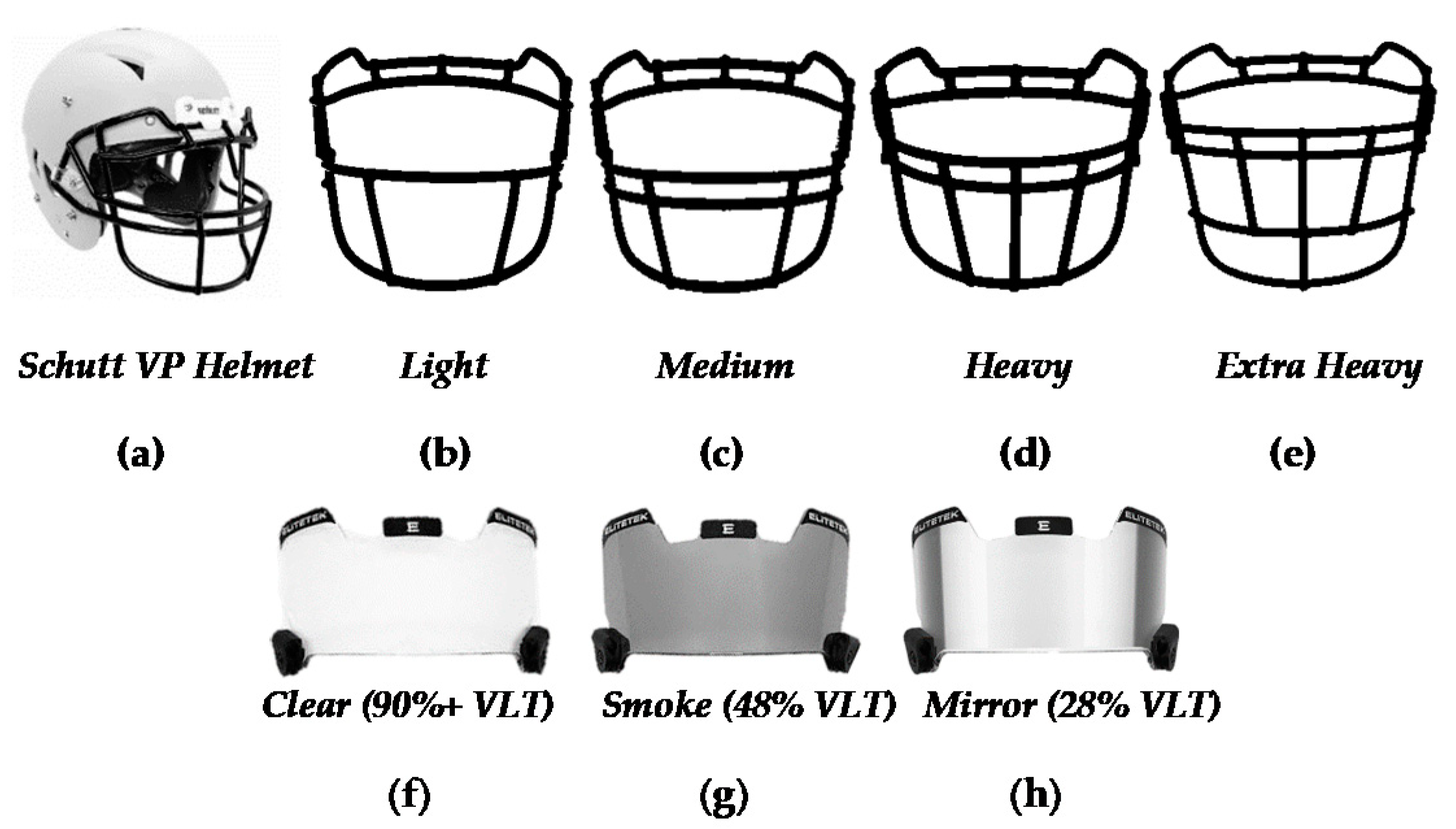This detailed black-and-white diagram of a SCHUTT (S-C-H-U-T-T) VP football helmet showcases various customizable options available for the helmet. In the upper left corner, there's a photograph of the helmet labeled “A,” complete with a basic face mask. Alongside this, the first row illustrates four different types of face masks labeled B through E that can be attached to the helmet, ranging from light to extra heavy protection. The light mask (B) has only a couple of bars protecting the chin, the medium mask (C) includes an additional horizontal bar for enhanced rigidity, the heavy mask (D) adds extra vertical bars, and the extra heavy mask (E) forms an almost grid-like structure for maximum protection, ensuring no ball could penetrate or damage the face guard.

The second row depicts three designs for visors, which are labeled F through H. These visors are designed to clip or snap onto the helmet, over the selected face mask. The clear visor (F) boasts a 90% VLT (Visible Light Transmission), the smoke visor (G) has a 48% VLT, and the mirror visor (H) provides a 28% VLT. The entire presentation, with its white background and monochromatic elements, is designed to aid in visualizing and selecting the preferred combination of helmet, face mask, and visor.